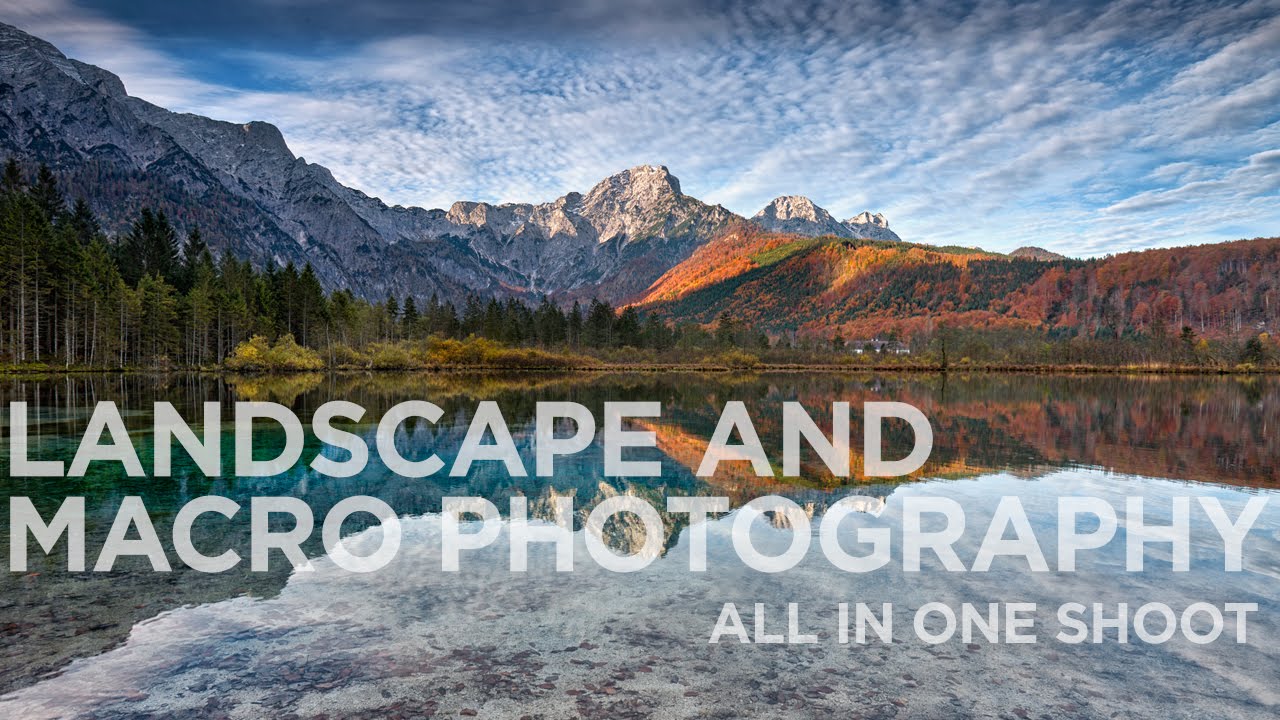A stunning digital photograph captures a breathtaking outdoor landscape set under a fairly blue sky, where clouds extend from the mountains like sun rays, suggesting intentional contrails. The background features a majestic mountain range, with the highest peaks dusted in snow and covered with patches of green. Towards the right, the terrain descends into a lower mountain range with earthy golden rust tones speckled with greenery. To the left, a dense forest of tall pine trees blends seamlessly into the scene, which includes smaller bushes and low grass as it transitions to the center.

The middle of the image showcases a wide expanse of a serene lake, reflecting the vibrant autumnal colors of nearby foliage—orange, yellow, and green—with an occasional hint of red. The tranquility of the water is disturbed by the choppy wake left behind by a passing boat, providing dynamic contrast. This exquisite vista is complemented by some buildings nestled amid the trees on the right bank.

The entire scene is illuminated in hues of white, blue, orange, and green, creating a vivid and almost surreal representation of a landscape that combines elements of macro photography. Despite its otherworldly beauty, the image claims realism, potentially depicting an exotic location in the Himalayas. The photograph prominently features the text "Landscape and Macro Photography, all in one shoot," emphasizing the blend of detailed close-ups and grand scenic views captured in a single frame.